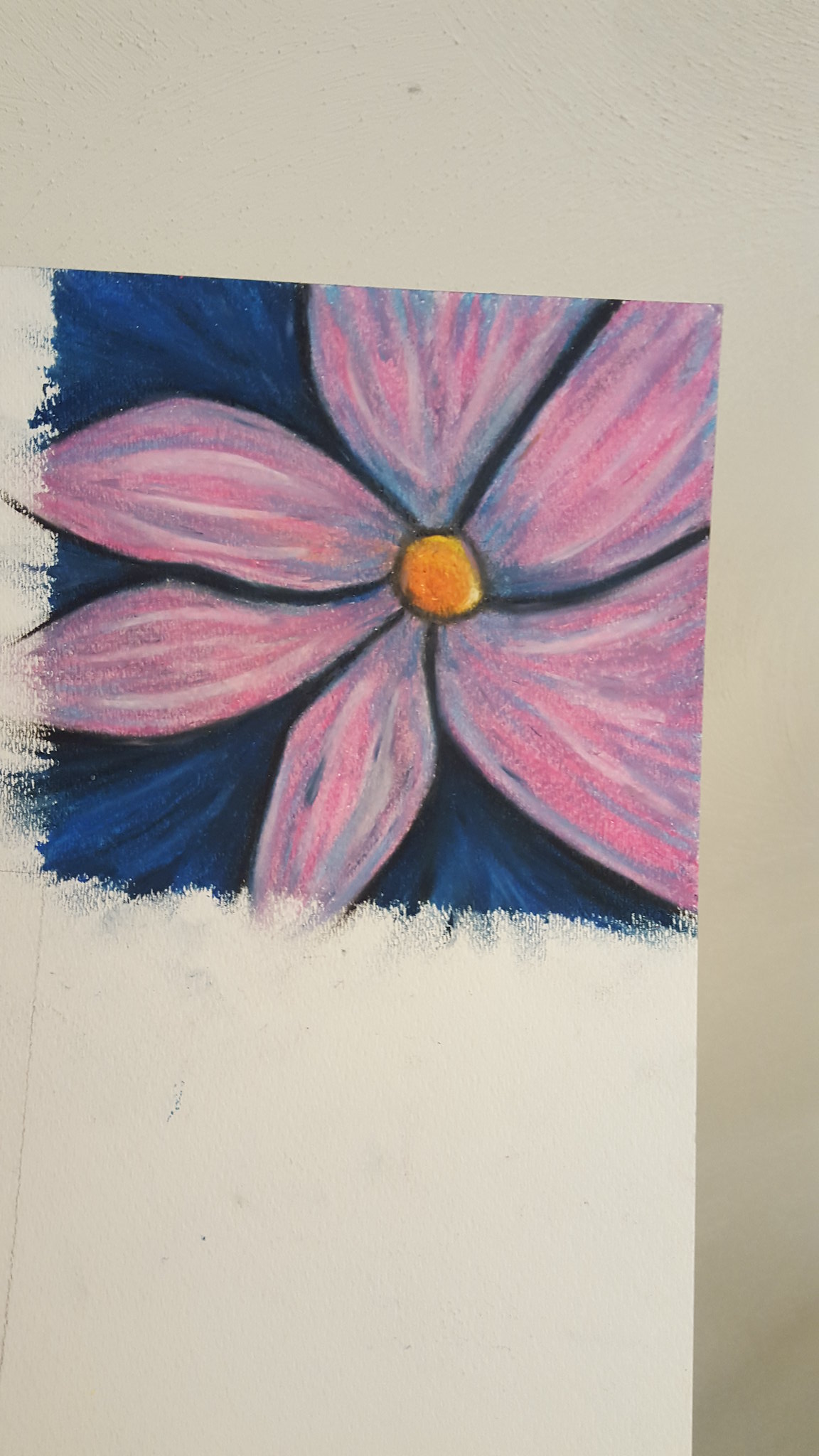The image depicts a childlike drawing of a flower situated on the upper right corner of a white piece of sketchbook-like paper, characterized by a textured, canvas-like look. The flower features a slightly irregular yellow circular center. Surrounding this center are six petals—three on the right, significantly larger and roughly double the width of the three smaller petals on the left. Each petal is ovular and rounded to a point at the end. The petals are predominantly pink, with some lighter pink and blue streaks, and are outlined in black. The background within the flower’s perimeter consists of alternating dark blue and black stripes. The entire artwork is positioned on a gray surface, and the lower half of the paper remains blank and untouched.